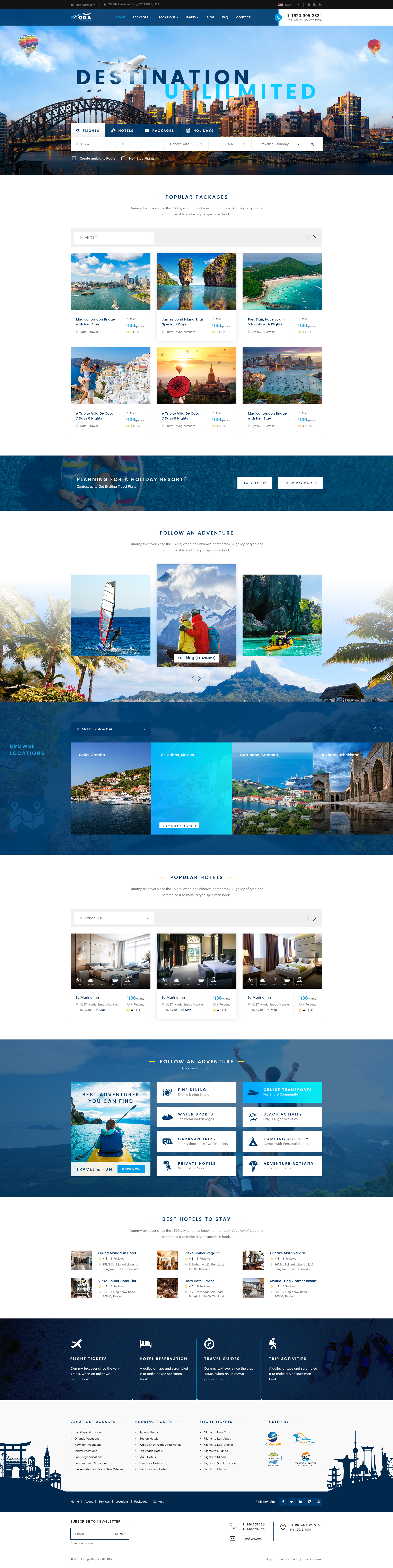The image features a detailed webpage layout for "Destination Unlimited." The page displays a vibrant city skyline with blue skies, scattered clouds, an airplane, and several hot air balloons hovering above. Highlighted sections include "Popular Packages," with visuals of four scenic water areas showcasing beaches, cliffs, and clear blue skies. One image captures a picturesque sunset adorned with additional hot air balloons and a person standing on a rooftop, gazing over a bustling city.

Further sections promote "Planning for a Holiday Resort," featuring palm trees, mountains, snowboarding, surfing, and kayaking activities. Another part presents a scenic city by the water, and "Popular Hotels" are showcased with images of three distinct hotel rooms.

The page inspires adventure with imagery of a person kayaking on serene blue waters, while another individual is seen in the background with arms outstretched, embracing the experience. Text highlights include "Best Places to Stay," "Flight Tickets," "Hotel Reservations," "Travel Guides," "Trip Activities," and "Vacation Packages."

Additional calls to action include booking options for flight tickets, noting trust by users, and an invitation to subscribe to their newsletter. The footer provides business details: a 2018 design theme, located at 7-5 Street Avenue, New York, New York 10011 USA, with contact number 1-811-920-3054 and email info@something.com. Options for help, sending feedback, and privacy policy information are also available.